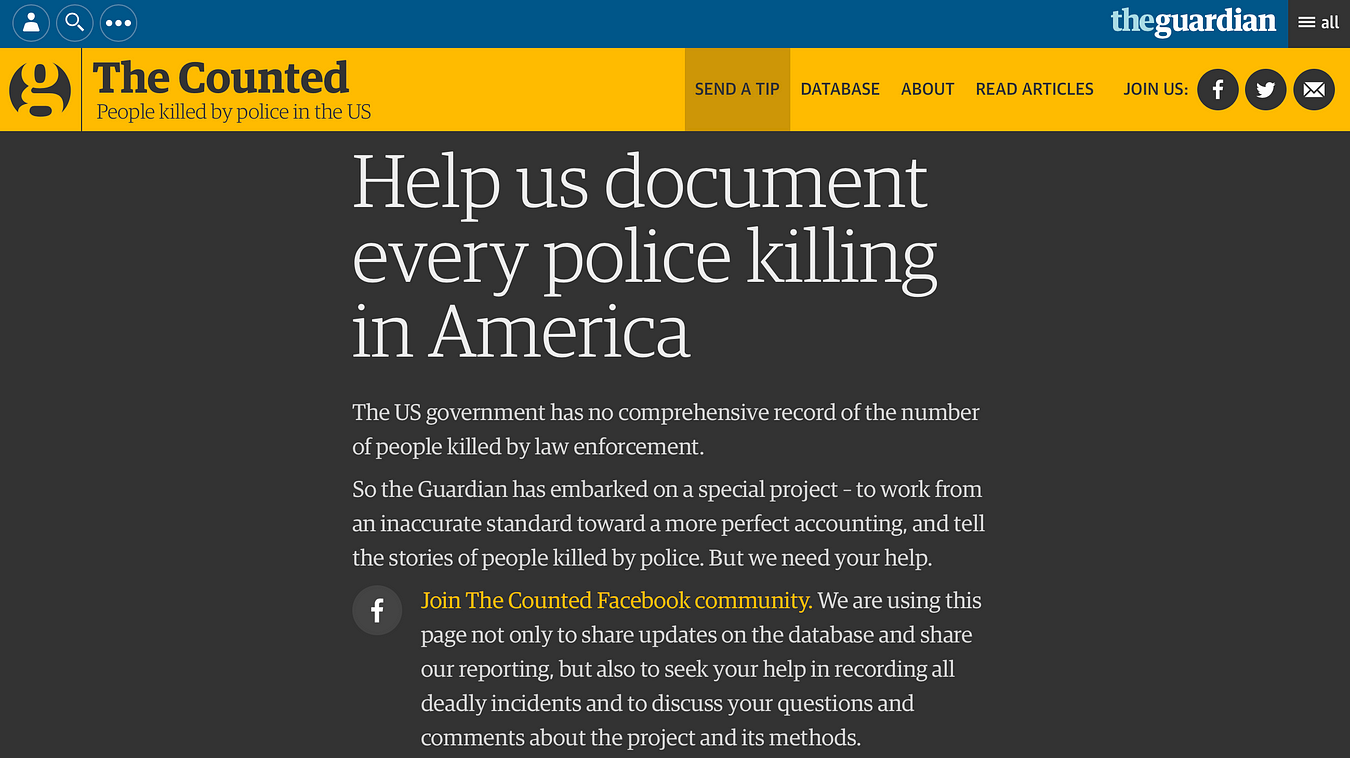The image displays the Guardian newspaper's website with a distinctive layout. At the top, a blue banner spans the width of the page. On the left side of this banner, there are small icons for logging in, searching, and a menu which likely provides additional options. The right side of the banner features the Guardian's logo and an all-pull down menu along with a small grey square.

Below this blue banner, a thicker yellow banner stretches across the screen. The left side of this banner is dedicated to "The Counted," a project that tracks people killed by police in the US. The right side offers several options: "Send a Tip," "Database," "About," "Read Articles," and "Join Us." The "Join Us" option is linked to social media platforms including Facebook, Twitter, and email.

The main section of the screen is dominated by a grey panel with prominent white text. The main heading reads, "Help Us Document Every Police Killing in America." Below this is a paragraph of text. Notably, the phrase "Join The Counted Facebook Community" is highlighted in yellow, and a Facebook link is situated to the left of this highlighted text.